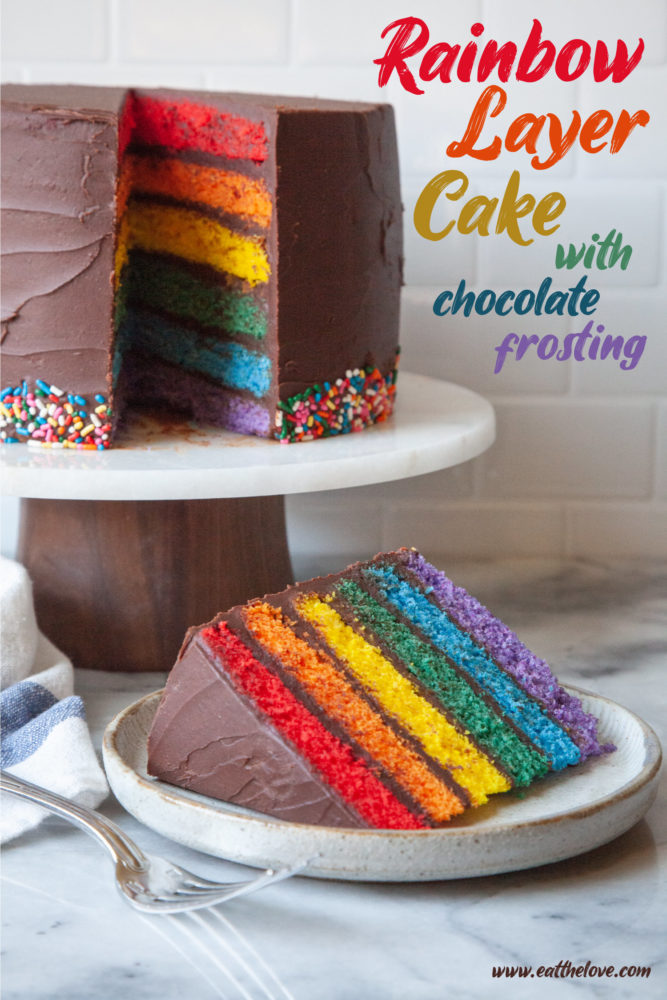This photograph captures a visually stunning rainbow layer cake with rich chocolate frosting, showcased on a sophisticated white marble cake stand with a brown wooden base. The centerpiece cake has one slice meticulously removed and placed on a shallow ceramic plate with a marbled pattern, accompanied by a silver fork resting on a marble countertop. The background reveals a white brick backsplash that complements the countertop. The cake itself features six vibrant layers in the colors of the rainbow: red, orange, yellow, green, blue, and purple, each separated by chocolate frosting. Additional details include a ring of rainbow sprinkles at the base of the cake. The text "rainbow layer cake with chocolate frosting" appears in corresponding rainbow colors at the top right corner, while the bottom right corner is marked with the website "www.eatthelove.com". The scene is subtly accented by a blue and white kitchen towel in the background, offering a touch of homeliness to the entire setup.